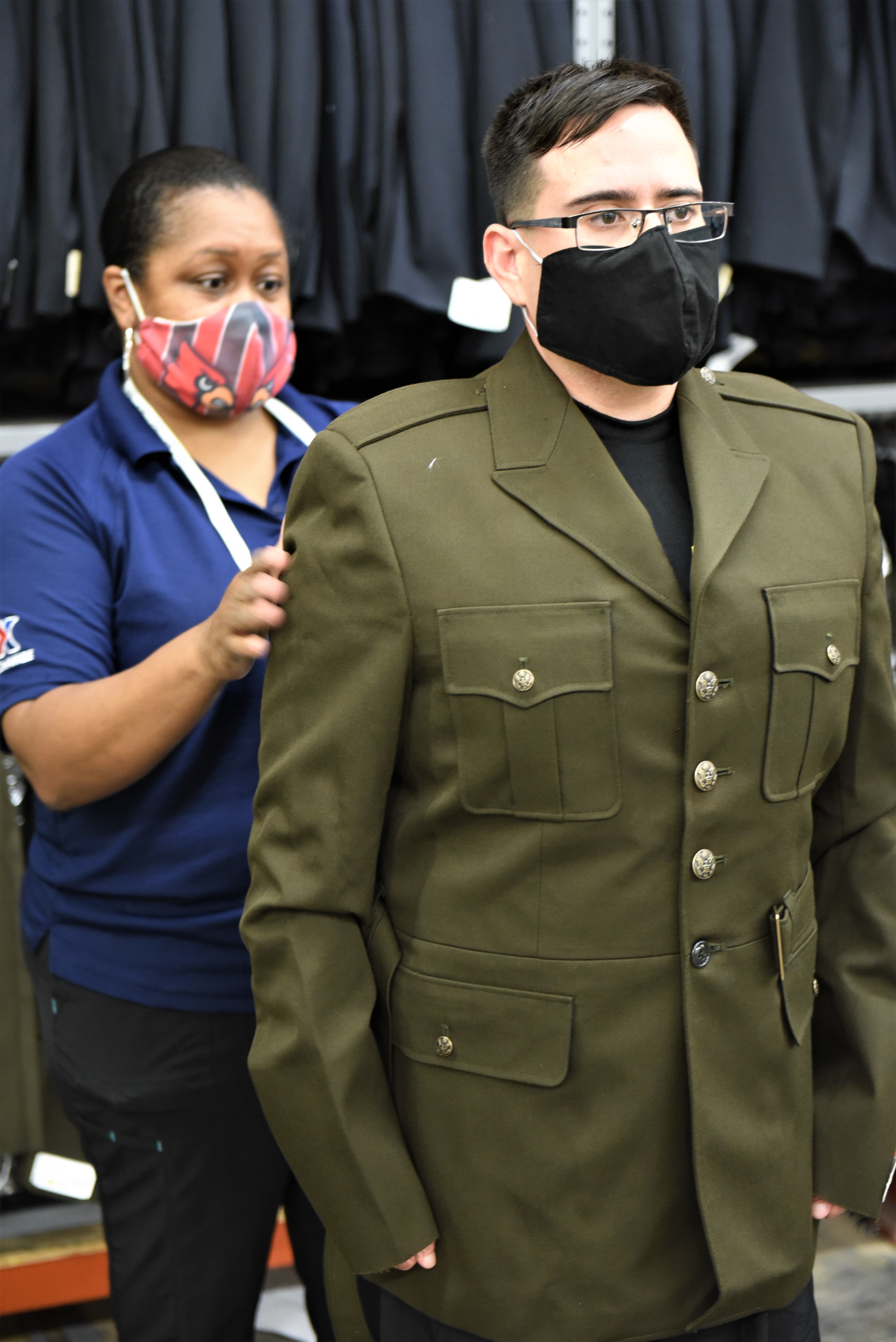The image depicts a man and a woman standing together, both wearing face masks. The man is dressed in a green, military-style jacket adorned with brass buttons and front pockets. He is also wearing glasses and a black COVID mask, looking straight ahead. Behind him stands a woman with her hair pulled back, donning a blue short-sleeved shirt with a collar and black pants. She is wearing a red mask with blue accents and has a tape measure around her neck. Her hands rest on the man's upper arms, as if she is adjusting or fitting his jacket. The background features a blue curtain and various clothing items hanging, suggesting a fitting room or a tailor shop setting.